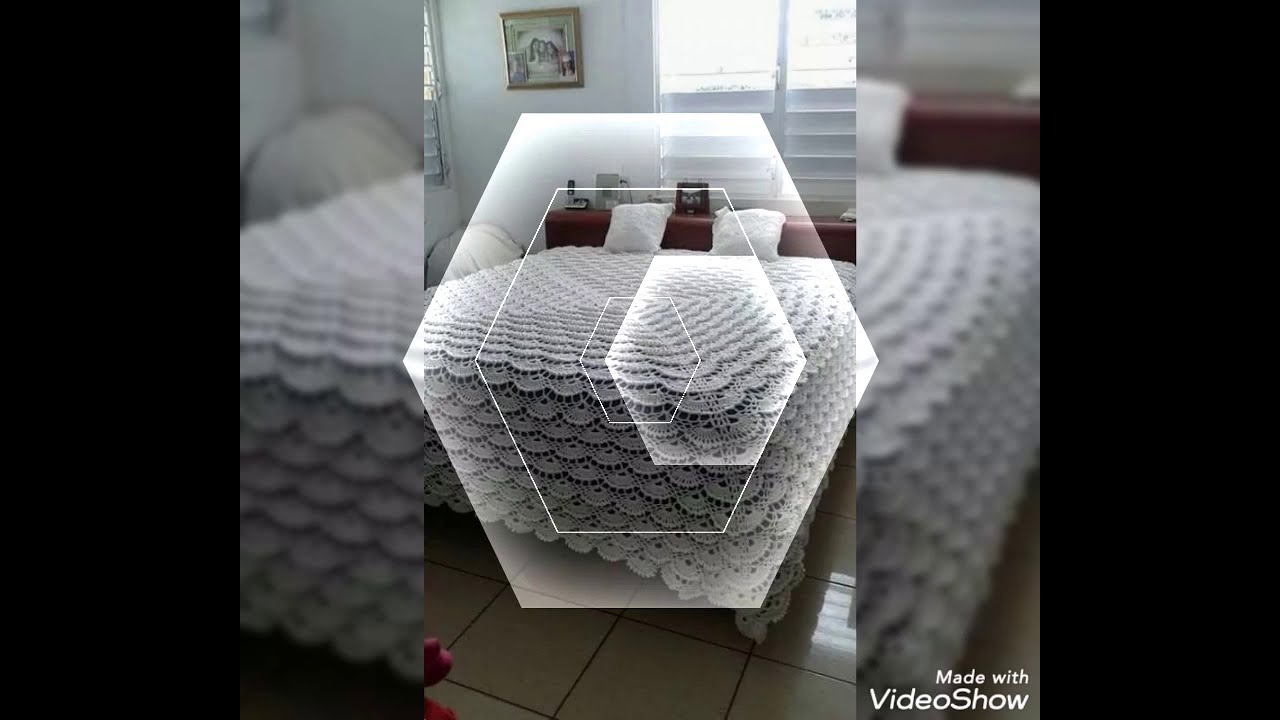This image is a complex, multi-layered composition reminiscent of a cubist painting. At its core, the photograph features a bed with a white ruffled comforter, two white pillows, and a brown headboard. The bed is the main subject, but the image is intricately superimposed upon itself multiple times, creating a visually confusing effect. The primary photo is cropped to a vertical portrait orientation and serves as the central focus. Surrounding this central image are progressively smaller hexagonal overlays, each one a closer view, allowing for detailed inspection of the bedspread's texture.

The entire composition is framed by thick black borders on either vertical side, creating a horizontal rectangular shape overall. Additional translucent and transparent panels are present, further adding to the layered effect and blending the boundaries between different superimposed images. The result is a fragmented yet cohesive portrayal of the bed and its setting, with varying levels of blur and clarity in different sections.

In the bottom right corner of the image, there is a watermark in white letters that reads "made with video show," confirming the use of specific editing software.